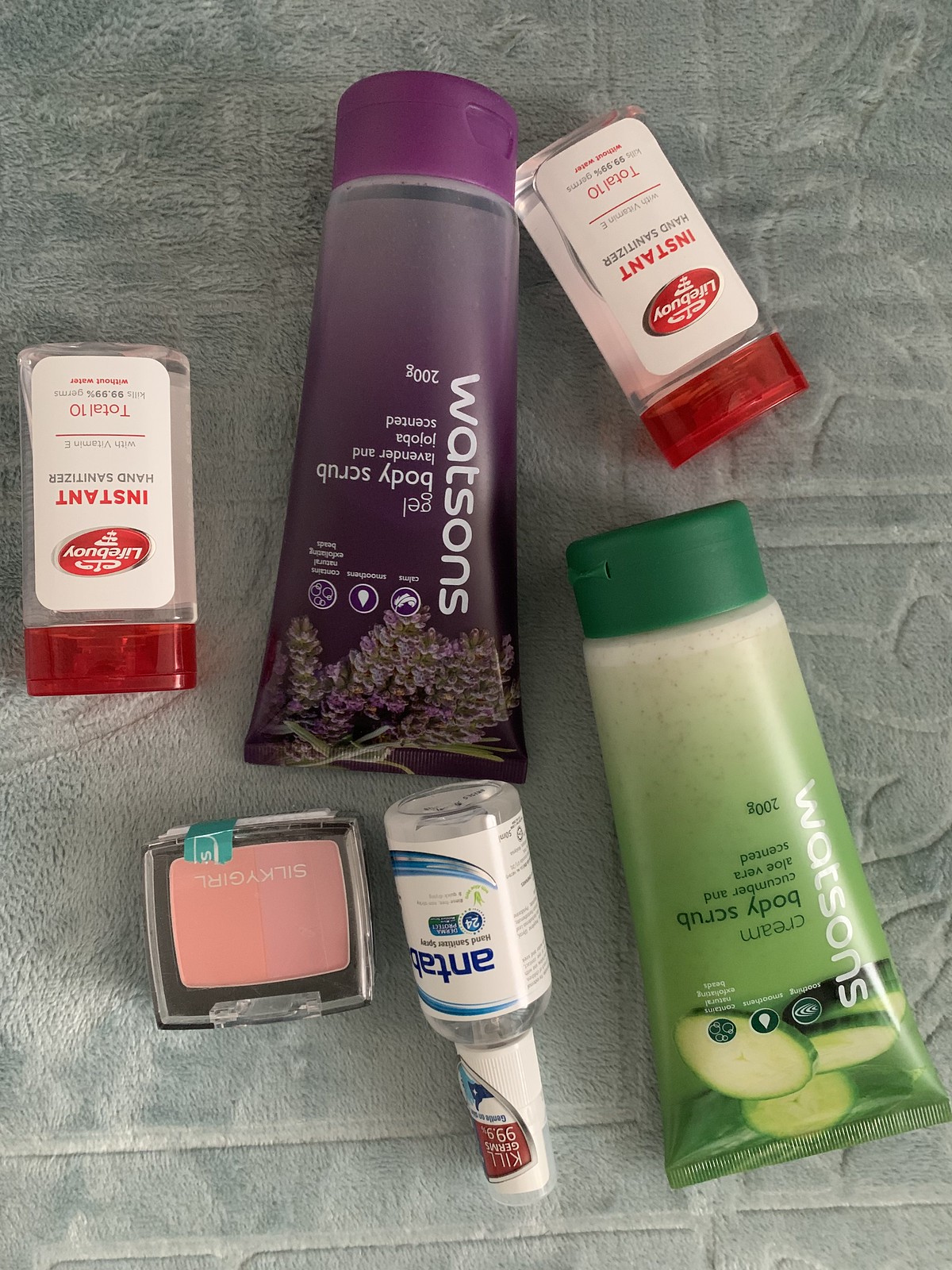The image depicts a grayish furred rug scattered with various skincare products. At the top center of the rug, there's a tube of body scrub labeled "Watsons," with part of the text shown upsidedown. The product details mention it is a lavender-scented body scrub weighing 200 grams and includes images of lavender plants and some circular icons with additional text. There is a purple cap on this tube.

On the left side of the image, there is an instant hand sanitizer bottle with a partially visible label indicating the words “life” and “something," featuring a red cap and a clear interior. A similar bottle appears at the top right, bearing the same characteristics and labeled “total 10.”

At the bottom right corner of the rug, another tube of Watsons body scrub is visible, this one cucumber and aloe vera-scented, also weighing 200 grams. The packaging displays cucumber slices at the bottom. Additionally, on the left-hand side is a silver bottle labeled with "kill germs, 99.9%,” a white cap, and a white label.

Further to the left, there is a clear container with a pink substance inside, branded "Silky Girl." Notably, many products appear upside down, suggesting the image was taken from an unconventional angle.